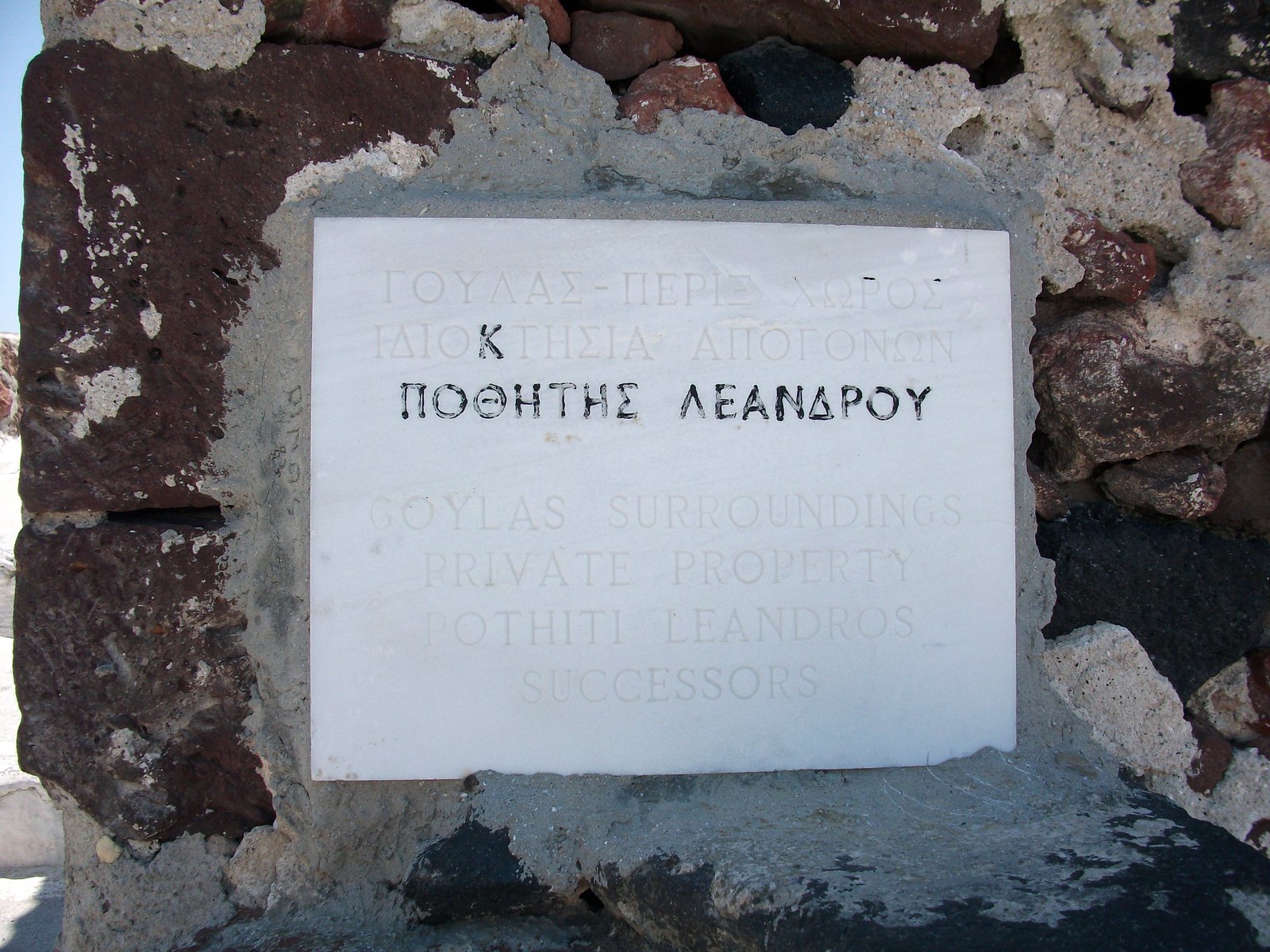In the photograph, we see an old stone wall constructed from irregularly shaped stones and bricks, predominantly in various shades of brown. The stones are cemented together with gray mortar. Attached to this wall is a white rectangular marble plaque. The plaque features imprinted text in a foreign language, likely Greek, with some segments of the text nearly faded and illegible. The majority of the text blends in with the white color of the marble, but there are distinct sections, particularly the third row down, where black lettering is still visible. The black letters include one that resembles the letter "K," which appears off-center to the left. The surface of the marble has a subtle glittery texture, adding a hint of gray and silver tones to its overall appearance.